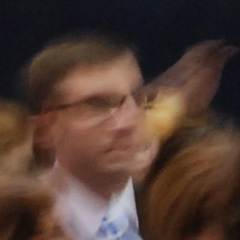This is a very low-resolution, color photograph taken in a dark room, rendering the background a complete black void. The image is notably blurry and captures a close-up shot from the neck up of an older Caucasian man. He is positioned amongst several indistinct figures, the tops of their heads barely discernible in the lower portion of the frame. The man, slightly turned to his right, has short light brown hair parted to the right, and wears a pair of glasses. He is dressed in a white collared shirt, a black suit jacket, and a blue tie. His expression appears upset. The overall poor quality, dim lighting, and blurred motion of the photograph create a ghostly, almost double-image effect.